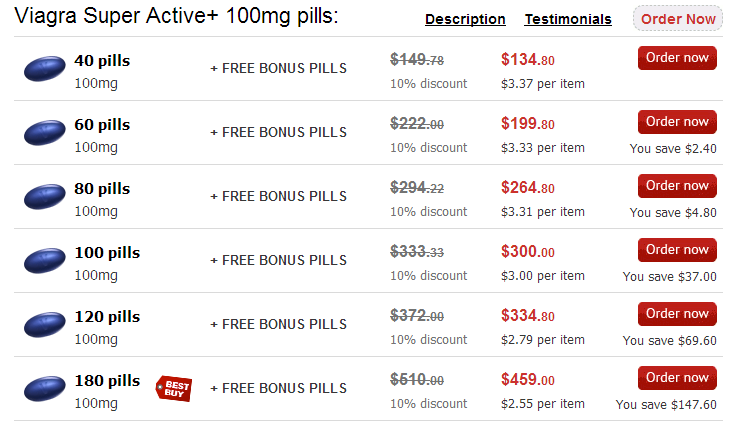The image depicts a webpage from an online pharmacy specializing in Viagra Super Active Plus 100 milligram pills. In the upper left-hand corner, there is a prominent large black font stating the product name. Directly to the right of this text, aligned horizontally from the middle to the right side, are three underlined sections: "Description," "Testimonials," and an "Order Now" button.

The webpage features a total of six rows, each offering different quantities of the pills alongside promotional bonus pills. The first row presents the option to purchase 40 pills, typically priced at $149.78, now available for a discounted rate of $134.80. An "Order Now" button is positioned on the right-hand side of this row.

The second row lists an option for 60 pills plus free bonus pills, originally priced at $222.00 but currently on sale for $199.80, indicating a savings of $2.40 compared to the previous option. This row also includes an "Order Now" button on the right.

The subsequent four rows continue to offer increased quantities of pills at progressively greater discounts, highlighting the promotional message: the more you buy, the more you save.